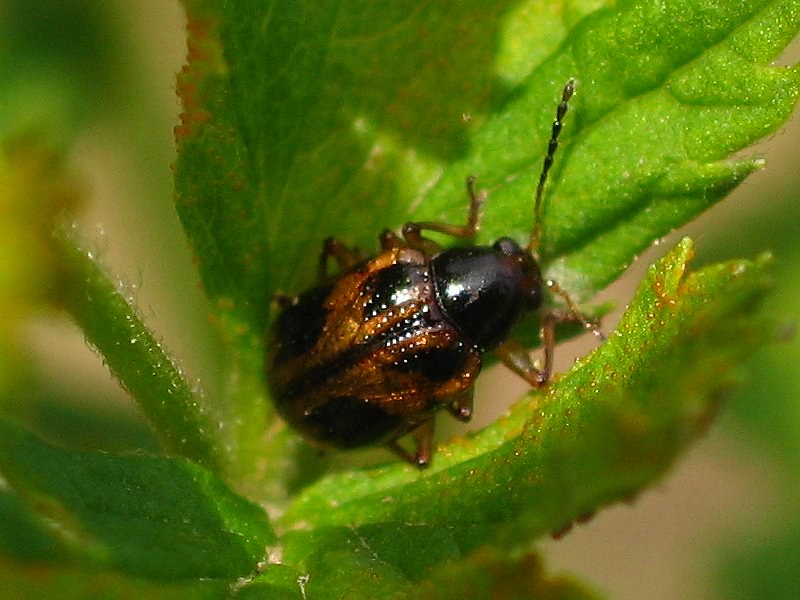A vivid close-up image captures a beetle sitting on a large, vividly colored green leaf, which appears to have gold specks and possibly a sticky texture. The beetle has a distinct and beautiful coloration with a dark body featuring gold and white speckles, and wings that are tinted in black and gold. It also has black markings, some orange hues, and possibly brownish tones. The beetle's several legs, likely six, are almost golden, and its antennae are clearly visible. This detailed photograph, although potentially unsettling for those who dislike insects, showcases the intricate beauty and unique appearance of the beetle with impressive clarity.